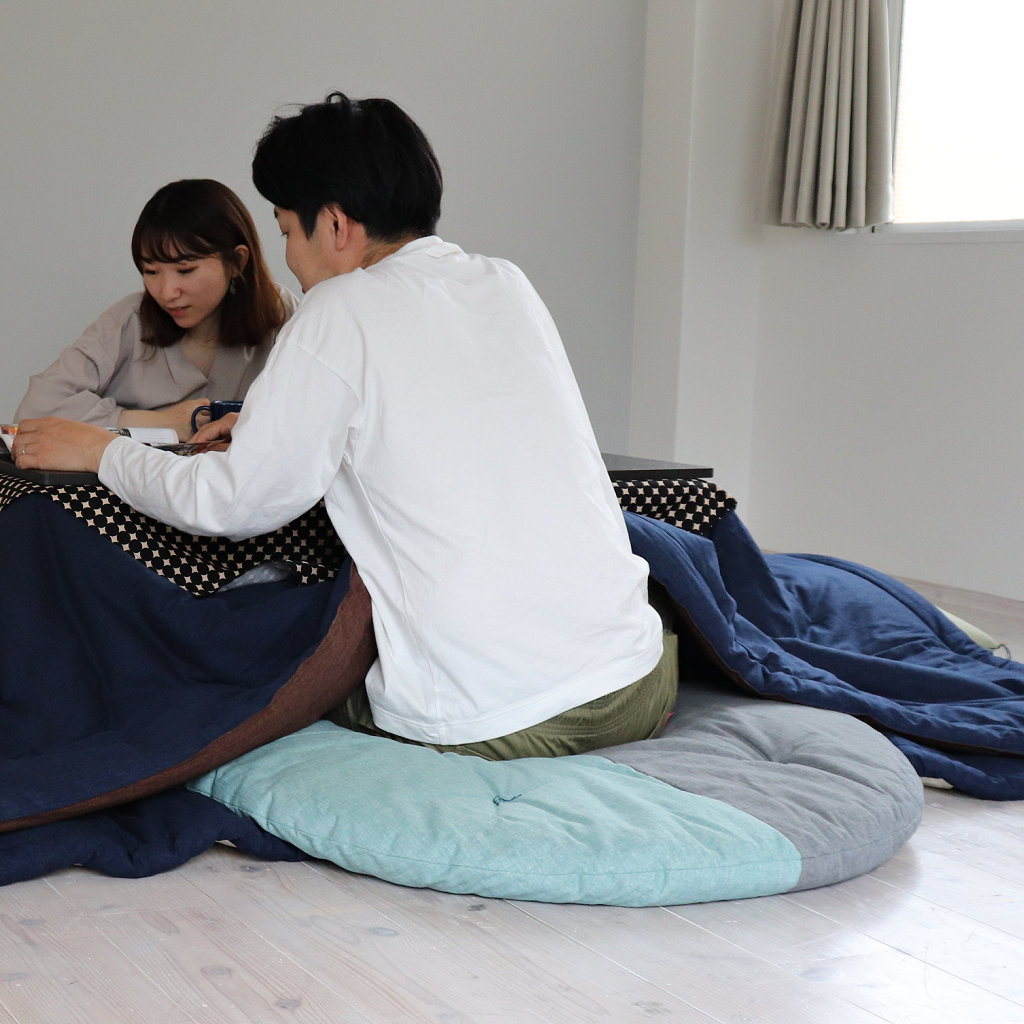In a nondescript room with crystal clear white walls and a vinyl plank floor that resembles light gray ash, a man and a woman, presumably Asian, are sitting beside a low table adorned with a dark navy and maroon tablecloth, which conceals a heater. They are on a thin cushion, half light blue and half gray. The man, wearing green pants with a long sleeve white shirt, a wedding ring on his left hand, is leaning over the table towards the woman. The woman, with shoulder-length brown hair and bangs tucked behind her ear, dressed in a beige shirt, is looking intently at an unseen object on the table. A white mug sits in front of her. The image, taken from a perspective that obscures what they are examining, instills a sense of curiosity and wonder. A window with a drawn-back curtain completes the serene setting.